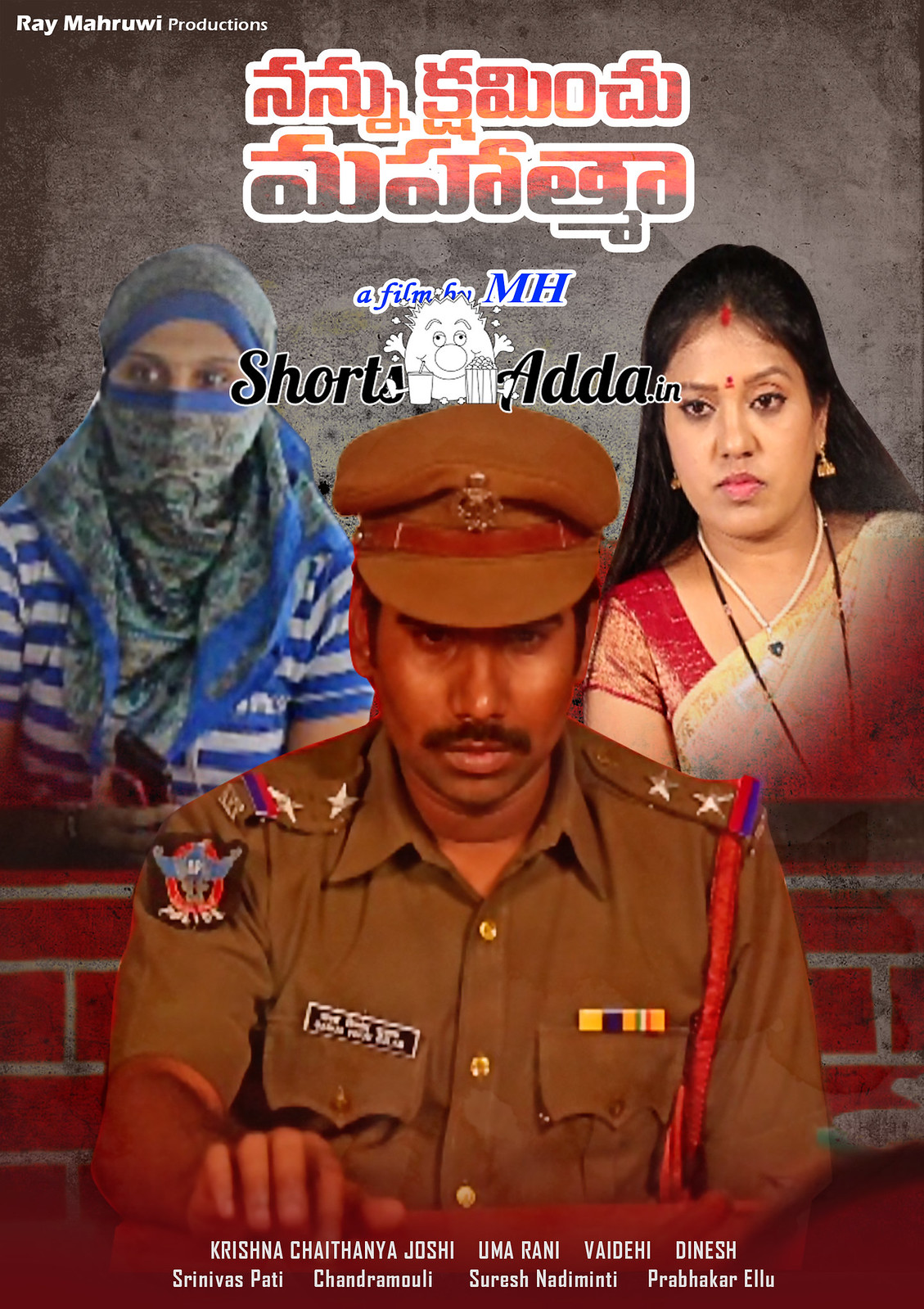The image resembles a movie poster with text in an unfamiliar language, possibly Arabic, at the top. The central title in a different language, featuring distinct alphabetical icons and an orange and deep gray color scheme, credits the film to M.H. Below the title, the poster showcases three East Indian characters against a brick wall background: a seated man in a military uniform complete with a brown hat, button-down shirt, epaulets, and various insignia, who appears to be either a policeman or an army sergeant with a mustache and a contemplative expression. Flanking him are two women; one on his left wears a blue and gray striped shirt, a gray turban-like mask, and a hat, while the other on his right dons a traditional sari, earrings, a pearl necklace, a sarong, and has a jewel on her forehead between her eyebrows. The bottom of the poster features a bar with different names, suggesting some sort of credits typically found on movie posters.